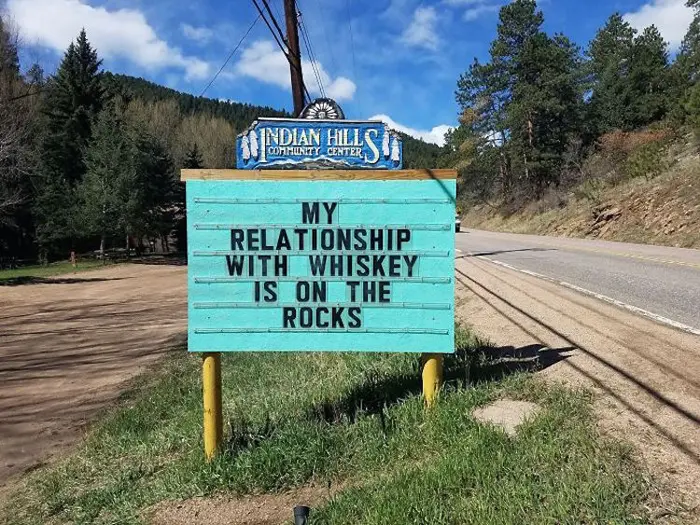The image captures a vibrant, detailed roadside scene in a remote, forested area far from the city. At the center of the composition stands a unique and humorous roadside sign sponsored by the Indian Hills Community Center. The sign, positioned between a paved road on the right and a dirt road on the left, is held up by two bamboo trunks and rests on a small grassy island. 

The sign itself is a color photograph in landscape orientation, featuring a turquoise background with black lettering that humorously reads, "My relationship with whiskey is on the rocks." Above this, a handcrafted sign in blue and white letters announces the "Indian Hills Community Center," adorned with a white radial half-circle design.

Behind the sign, tall pine trees and a tree-covered hill add to the natural, wilderness atmosphere. The scene is bathed in sunlight, casting distinct shadows from overhead power lines, suggesting a clear, bright day. The overall style is one of photographic representationalism, capturing the charm and quirks of this unusual community sign in a realistic and detailed manner.